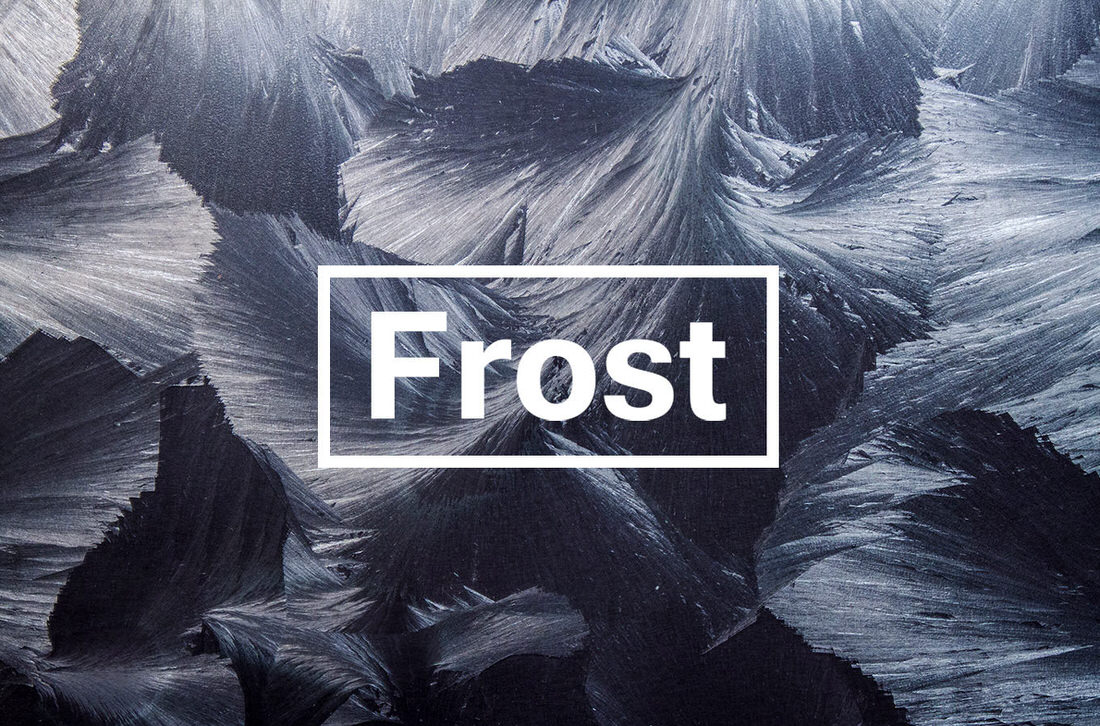The image showcases an abstract, computer-generated artwork featuring a mix of black, gray, and white paintbrush strokes arranged in a wavy, textured pattern reminiscent of icy leaves or frosty landscapes. This artistic design dominates the entire frame, with darker shades concentrated at the bottom slowly transitioning to lighter shades toward the top, enhancing the frost-like impression. Central to the composition is a transparent white rectangular outline that encloses the word "FROST" in bold, white text, which is likely indicative of a brand name. The overall effect of the image evokes a sense of winter and cold, amplified by the monochromatic color scheme and the textured, wave-like brush strokes.